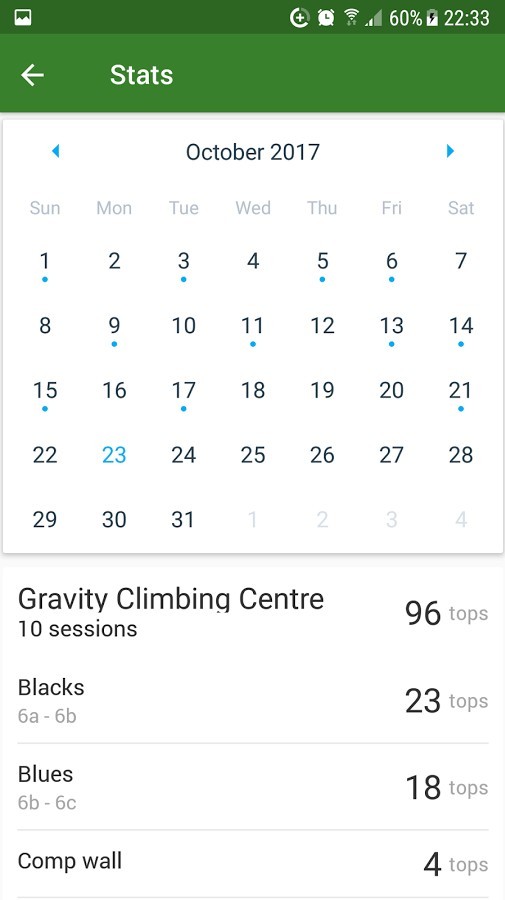In the image, we see a detailed view of a digital calendar interface set to the morning of October 17, 2017. At the top of the screen, a green rectangle houses several icons: a plus icon for adding events, a clock icon, full WiFi signal, a partially filled signal bar indicating moderate cellular reception, a battery level at 60%, and the time displayed as 22:33. Below these icons, there's a left arrow followed by what appears to be a navigation or menu icon.

Below the header, the days of the week are displayed: Sunday, Monday, Tuesday, Wednesday, Thursday, Friday, and Saturday. Small blue dots mark specific dates: the 1st, 3rd, 5th, 6th, 9th, 11th, 13th, 14th, 15th, 17th, 21st, and the 23rd, which is highlighted in blue, indicating an active or selected date.

Further down, the calendar contains text entries detailing events and sessions at a climbing gym named "Gravity Climbing Center." The calendar notes "10 sessions, 96 tops," "Black: 76A dot 6B, 23 tops," and "Blue: 6B dot 6C, 18 tops." Additionally, "Comp 1" is noted with "4 tops."

The background of the calendar is white, and it lists "Scott Gibson" repeatedly, implying that the calendar belongs to or is set up by Scott Gibson.

Overall, the image depicts a highly organized and detailed schedule, particularly focused on climbing sessions and associated statistics at the Gravity Climbing Center.